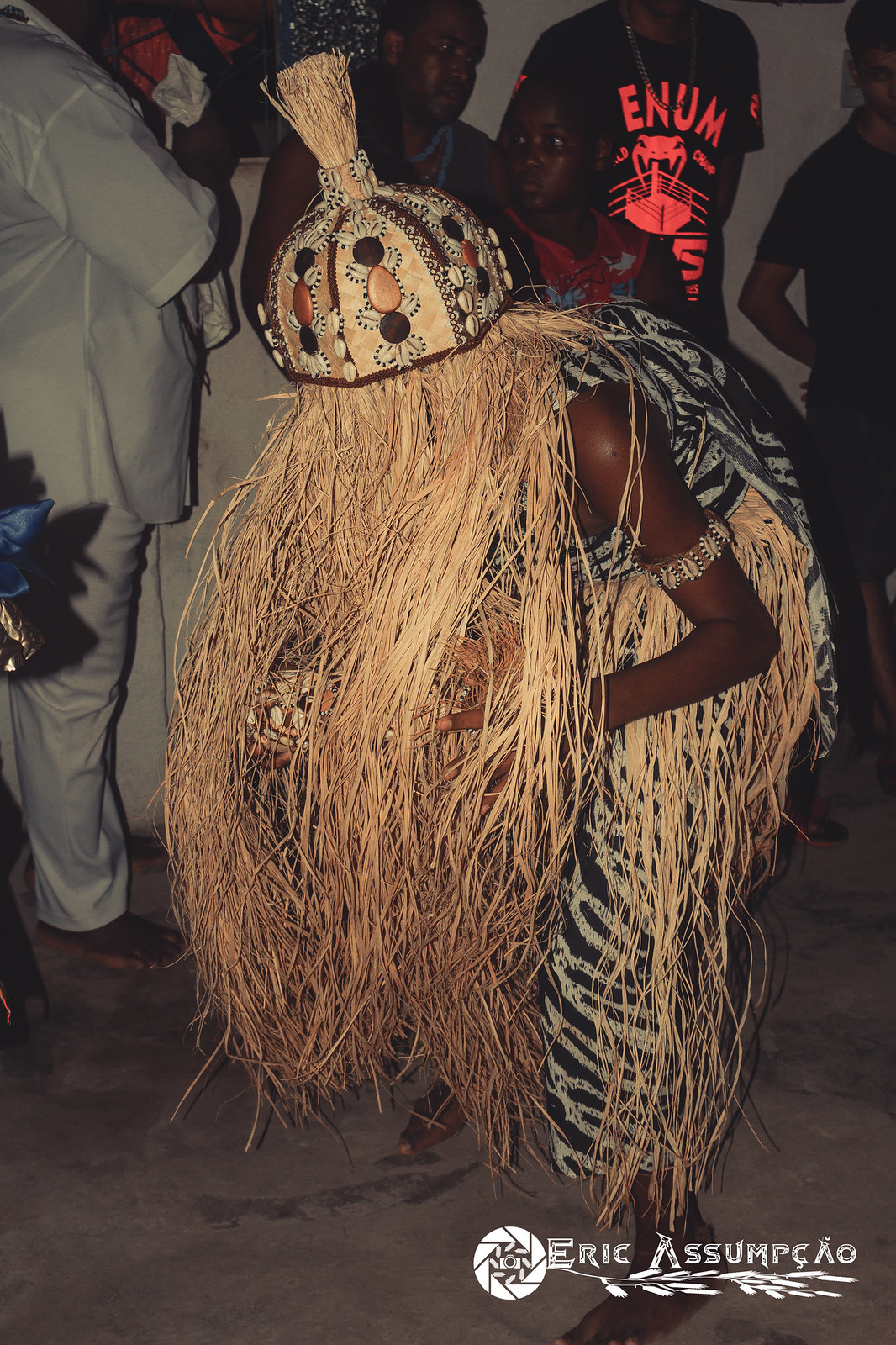The photograph captures a striking image of an individual dressed in a traditional tribal costume, seemingly participating in a performance or ritual. The scene is rich with cultural elements; the central figure is adorned in a black and white striped garment, resembling zebra stripes. Visible parts of the person include a bare arm with an upper-arm bracelet and bare feet. The headpiece of the costume is particularly elaborate, resembling an upside-down bowl adorned with brown and white shells and featuring an abundance of long, yellowish dried grass stalks that cascade down to the ankles, obscuring the person's face and adding a dynamic flow to the attire. The individual appears to be crouching slightly, possibly engaged in a dance, holding an indistinct object. In the background stands another person dressed in a modern white short-sleeved shirt and long white pants, along with several other onlookers whose faces are mostly indistinct. The photograph is credited at the bottom to Eric Asumpkayo, accompanied by a logo and a wheat stalk symbol.